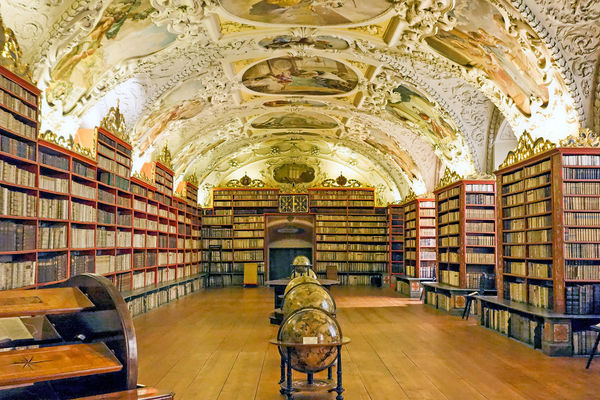The image captures the stunning interior of a grand library with an artistically domed, white ceiling adorned with elaborate oil paintings depicting men and women, some in oval portraits surrounded by intricate artwork. The room, bathed in natural light, features tall, redwood-colored bookshelves lining the left wall and splitting vertically at the back wall to accommodate what appears to be a fireplace. The right-hand side includes shorter sections of shelves interrupted by doorways. Dominating the center of the room are several large, yellow globes encased in wooden structures, resting on dark brown feet. In the foreground, a wooden desk stands to the left, while the entire floor is made of wood, adding to the room's warm ambiance.